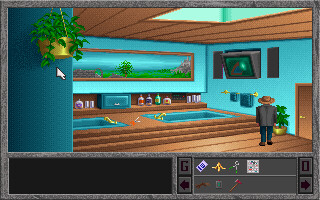This image is a screenshot from a computer video game, which is evident from the mouse cursor positioned three-quarters up on the left side of the screen. The central focus of the scene is a character wearing a cowboy hat, distinguished by the absence of any discernible facial features. This character is clothed in a large grey sports jacket, blue jeans, and brown shoes, lending a retro vibe reminiscent of the 1970s.

The setting appears to be an upscale spa or sauna, featuring a wooden floor and various bath or hot tub installations. The bottom right corner showcases a luxurious atmosphere, complete with a modern-looking TV and a large skylight that illuminates the room. The room is adorned with several plants, including one right beside the entrance at the bottom right and another hanging in the top left foreground.

A large painting of a rural scene decorates the wall, enhancing the rustic yet sophisticated ambiance. Numerous bottles are scattered around, likely containing chemicals or additives meant for the baths or hot tubs. Spanning the very bottom of the image from left to right is a game menu and inventory bar, indicating the player's available items and character options.